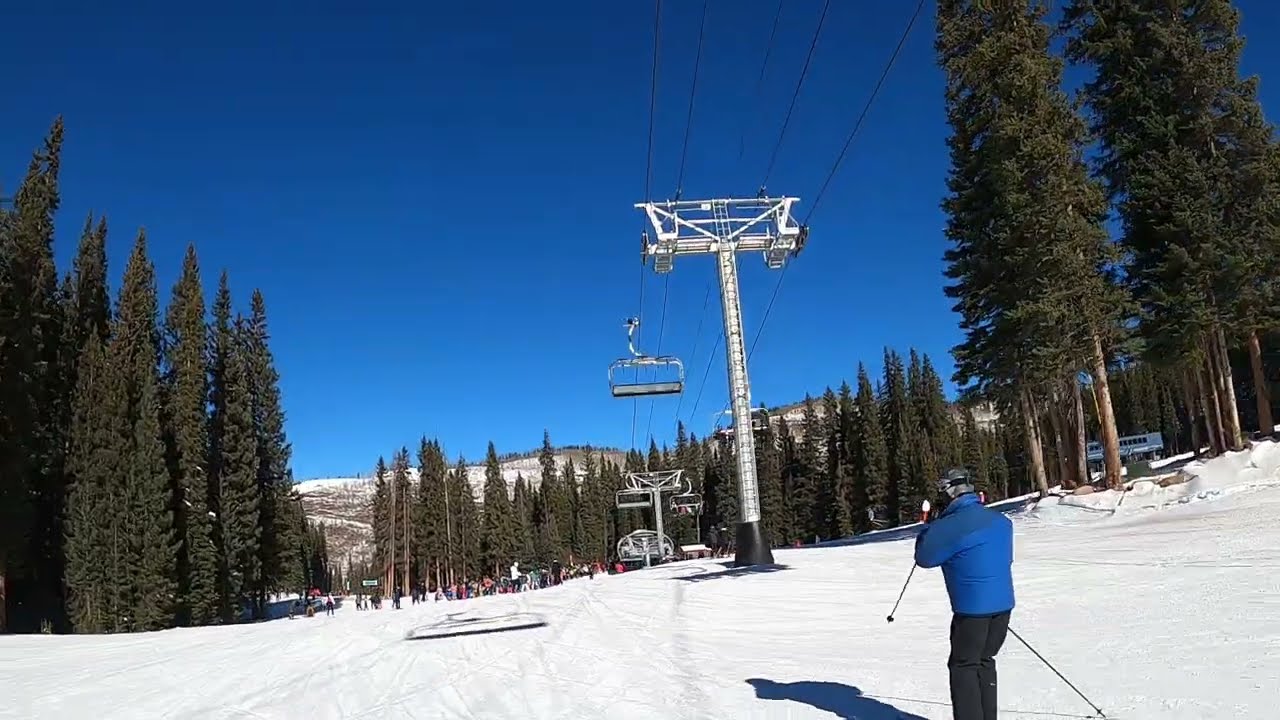This is a captivating photograph of a snow-covered mountain filled with vibrant winter activity. In the foreground, a skier dressed in a blue jacket and black pants is seen from behind, holding ski poles as they descend the slope. Surrounding the skier are tall, green pine trees that stand starkly against the white snow. Above the skier, white ski lifts span from the front to the back of the image, carrying numerous people up the mountain. To the right, there is a distant sign, though its details are indistinguishable. Numerous tiny figures and a line of people are visible near the base of the ski lifts, waiting for their turn to ascend. The background reveals additional snow-covered peaks, all beneath a perfectly clear, blue sky.